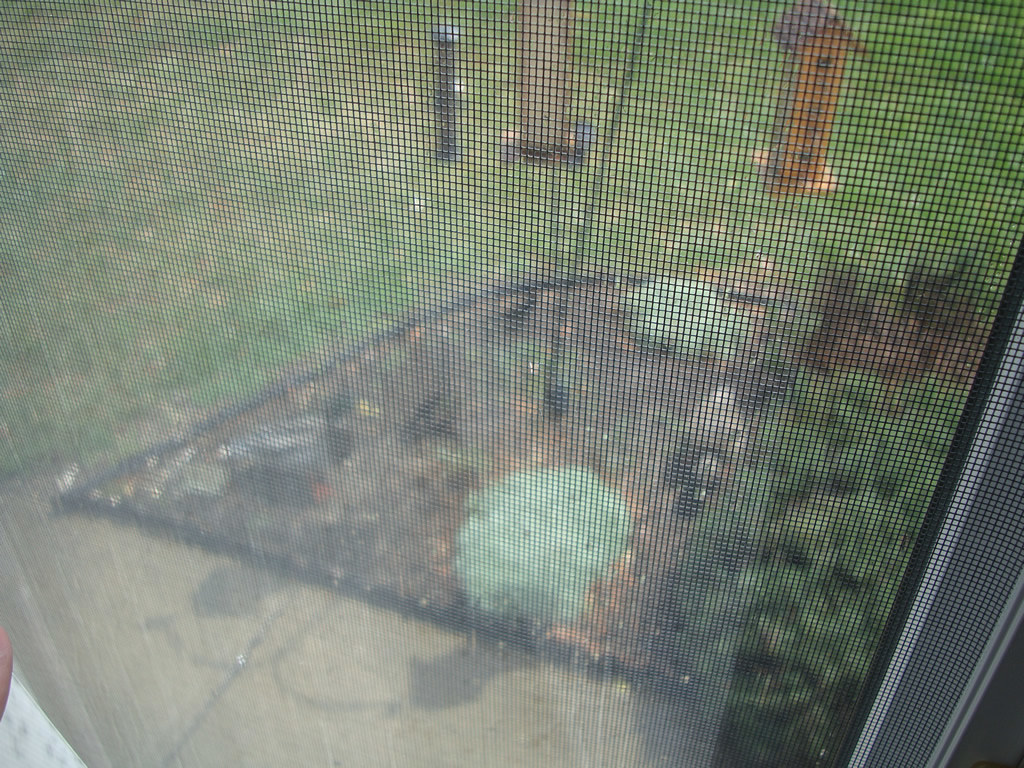The photo, taken through a screen door, showcases a backyard scene. The yard features a sectioned-off garden bed with decorative plants and bushes, some of which are white and green. The manicured grass borders a rounded-off dirt area with a few large gray rocks. A wooden birdhouse with an angled roof hangs prominently in the background, accompanied by at least one other bird feeder. The shadows of these birdhouses and feeders are cast on the ground, highlighting the sunny conditions. In the lower left corner, the image captures what appears to be part of a finger, adding a human element to the scene. Additionally, there is a long tube-like structure in the middle of the garden, though its purpose remains unclear. A hint of white trim from the screen door border is visible, completing the detailed view of the outdoor area.